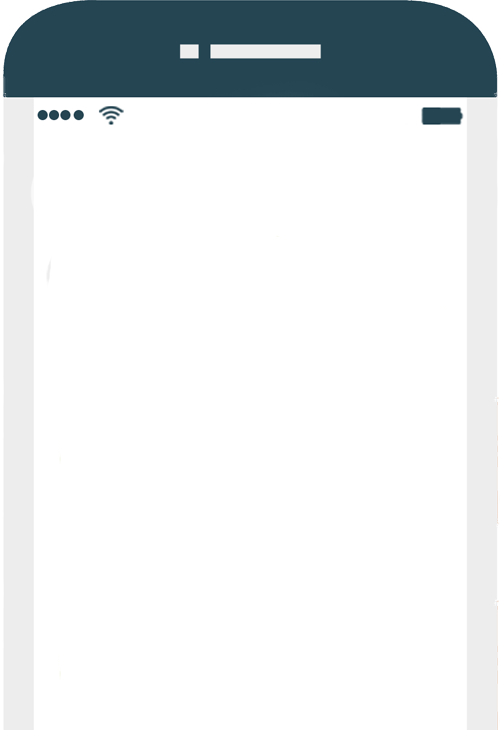The image depicts a portion of what appears to be a simplistic, clip-art style representation of a smartphone, likely an iPhone, given its distinct rounded edges and recognizable interface elements. At the top of the image, the phone’s rounded edges are clearly visible, characteristic of an iPhone design. A gray circular area at the top center of the phone likely represents the earpiece or proximity sensor. Near this gray circle is a small gray square.

Inside the phone's screen area, in the upper left corner, four dots are arranged in a square pattern, possibly symbolizing a signal or indicator light. Adjacent to these dots is a familiar Wi-Fi icon, suggesting network connectivity. Further to the right, a fully charged battery icon is displayed, indicating the phone has ample power. The gray borders on the left and right sides of the phone are slightly thicker, framing the screen and extending downwards. However, the image ends abruptly before revealing the bottom portion of the phone, which may typically include elements like the microphone or speaker grills.

Overall, the image serves as a rudimentary, large-scale visual designed perhaps for prototyping or testing purposes, with emphasis on basic visual elements rather than a fully detailed render.